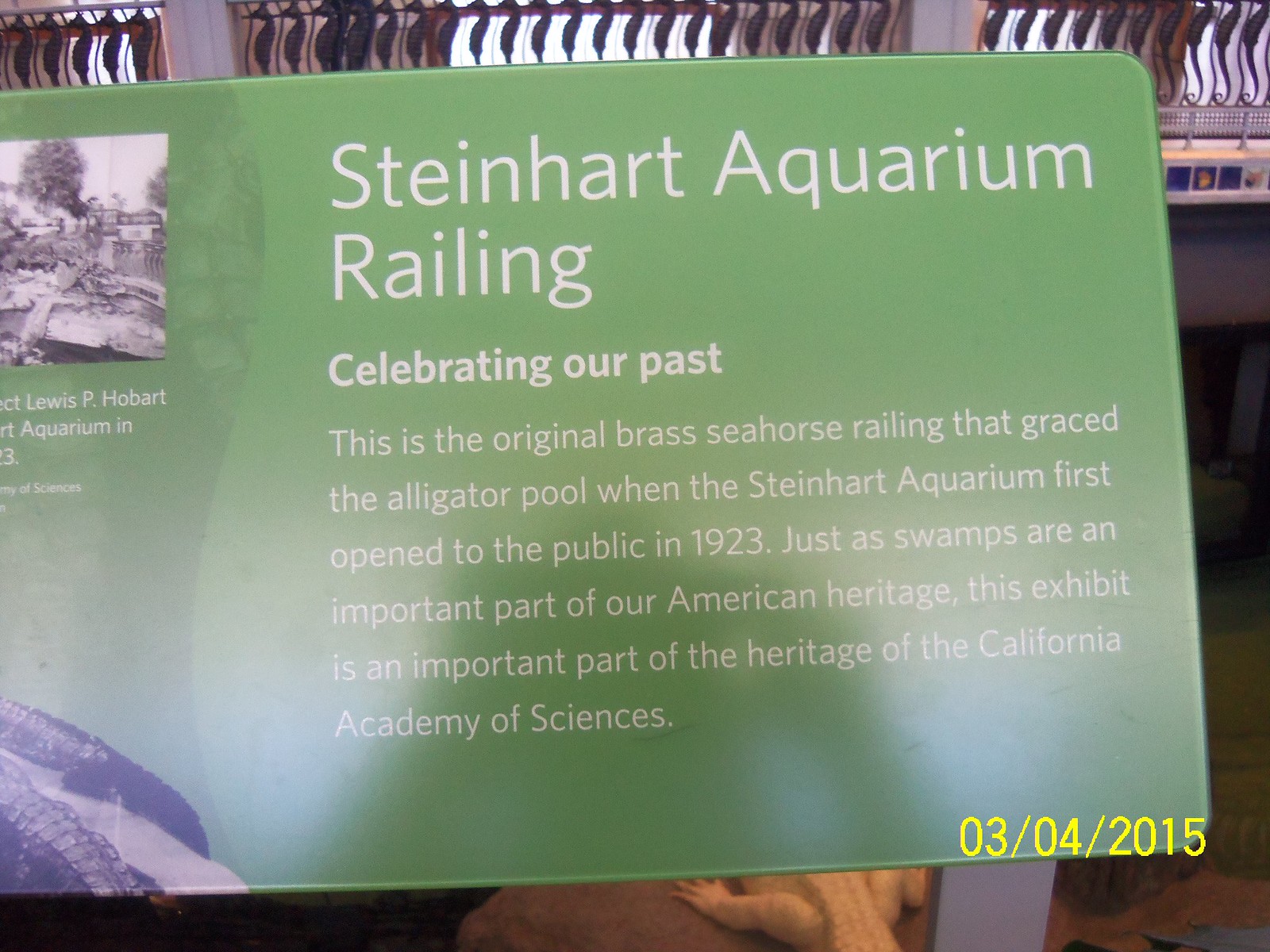This photograph captures an informational plaque commemorating the Steinhardt Aquarium Railing. The plaque, which features white text on a green background, reads: "Steinhardt Aquarium Railing. Celebrating our past, this is the original brass seahorse railing that graced the alligator pool when Steinhardt Aquarium first opened to the public in 1923. Just as swamps are an important part of our American heritage, this exhibit is an important part of the heritage of the California Academy of Sciences." To the left of the plaque are partially visible black and white photographs. Below, partially visible behind the plaque, is an albino alligator with only its back legs and tail showing. Additionally, in the background, you can see the brass seahorse railing mentioned on the plaque, partially obscured. The date the photo was taken, "03-04-2015," is noted in yellow text at the bottom right corner of the image.